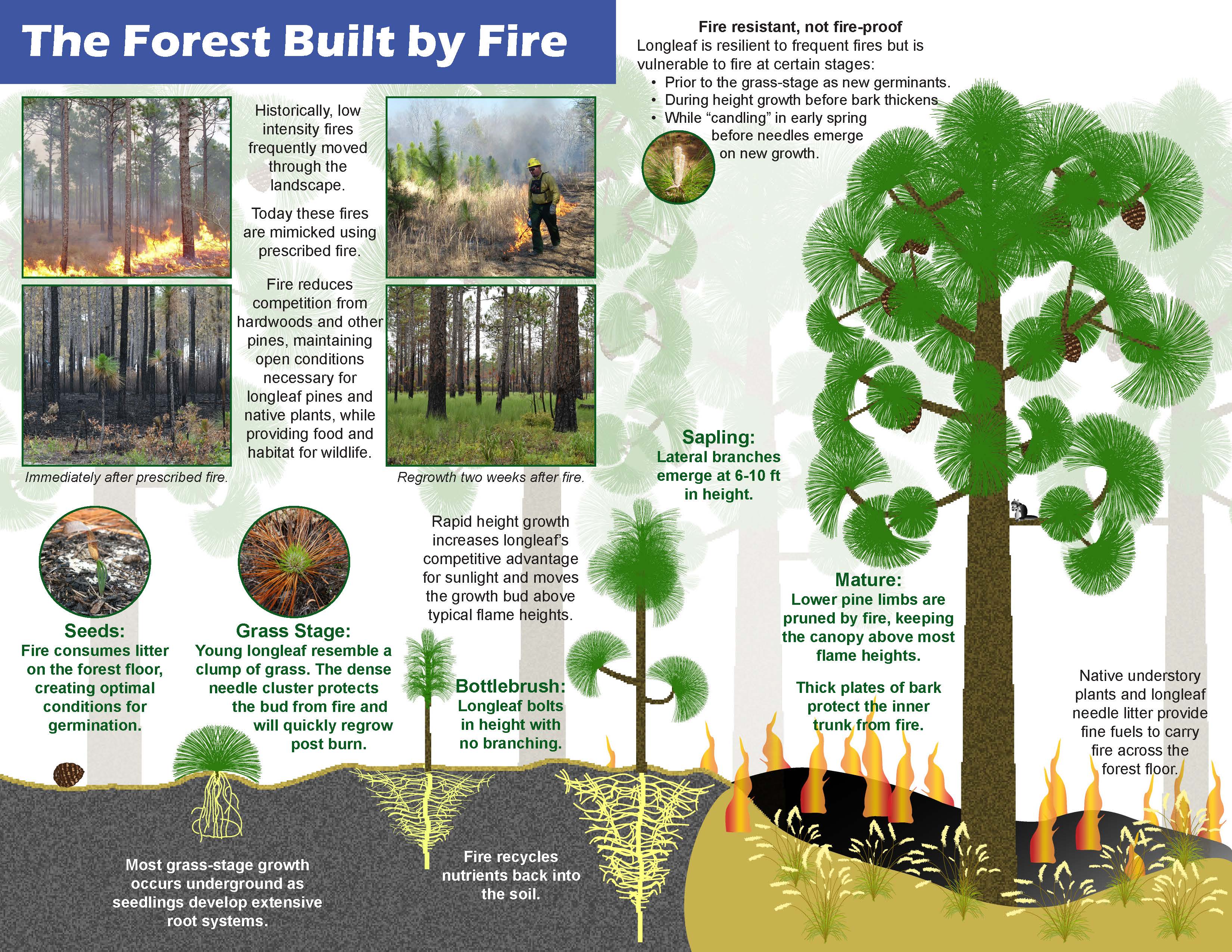The image, titled "The Forest Built by Fire," features a detailed diagram and an explanatory narrative situated on a blue border at the top left-hand side. In bold white letters, it explains how historically low-intensity fires frequently moved through the landscape and are now mimicked using prescribed fires. 

There are four sequential images at the top left illustrating the fire management process. The first image shows the initial fire moving through the trees, the second depicts a professional firefighter monitoring the fire, the third highlights the immediate aftermath of the fire, and the fourth demonstrates the regrowth of vegetation two weeks later.

Below these images, the accompanying text details how fire reduces competition from hardwoods and other pines, maintaining the open conditions necessary for the growth of longleaf pines and native plants. This fire management also provides food and habitat for wildlife.

To the bottom left, an additional diagram shows a gray ground with green saplings emerging. Adjacent to this, on the right, two circles labeled "seeds" and "grass stage" outline how fire consumes litter on the forest floor, creating optimal conditions for seed germination. It further explains that young longleaf pines resemble a clump of grass, with dense needle clusters protecting the bud from fire.

Another notable section highlights that while longleaf pines are fire-resistant, they are not fire-proof, and their vulnerability changes at different growth stages. The rapid height growth of longleaf pines gives them a competitive advantage for sunlight, moving them above typical flame heights, and the most significant growth occurs underground as seedlings develop extensive root systems. Additionally, native understory plants and longleaf needle litter provide the fine fuels necessary to carry fires across the forest floor.

Overall, the image presents a comprehensive overview of forest fire management, its benefits for longleaf pine ecosystems, and the natural regenerative processes driven by fire.